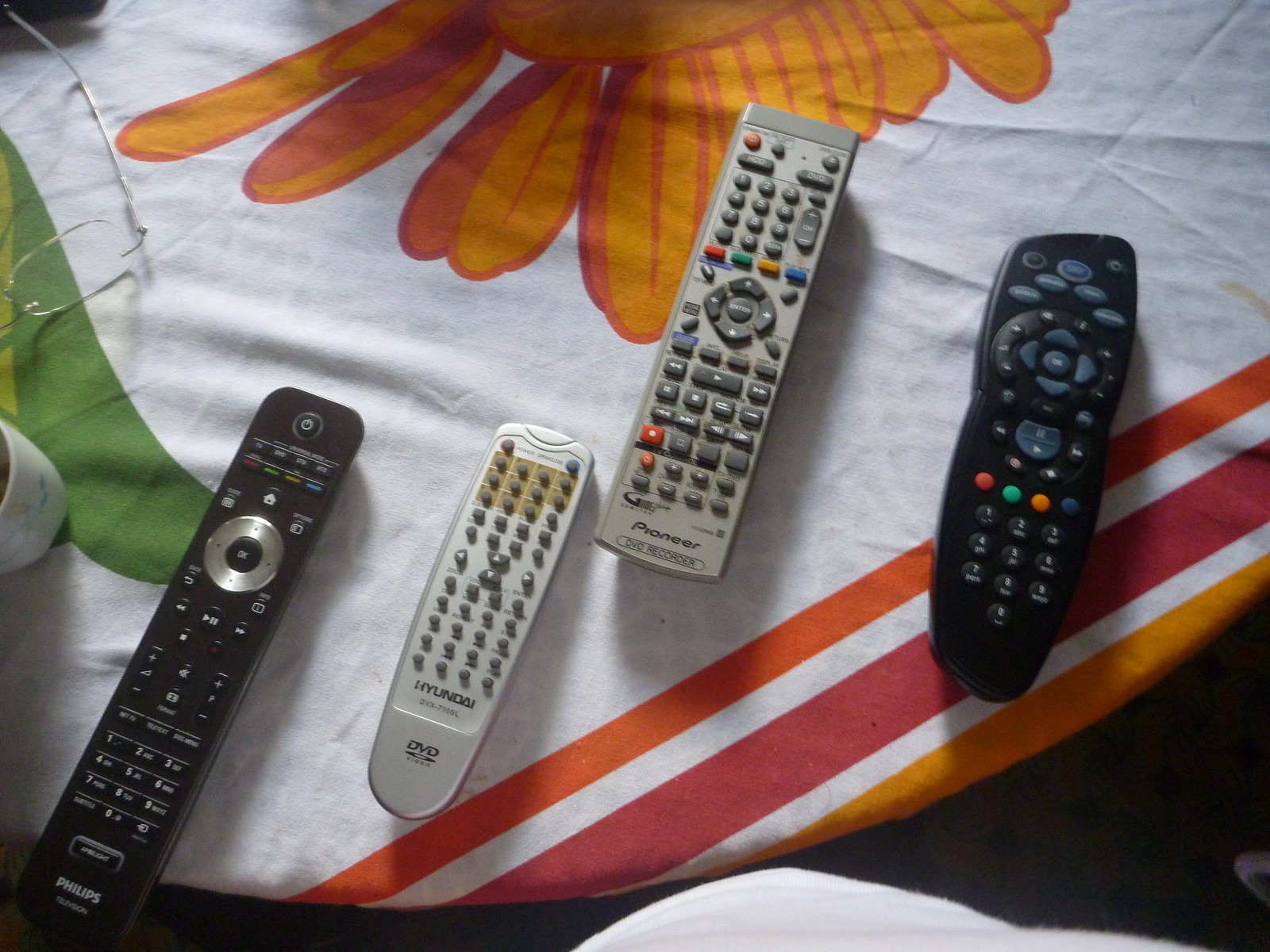In the image, there are four television remotes placed on a table covered with a patterned tablecloth. The tablecloth appears to be designed for a rectangular table but is being used on a small, round table, leading to some of the pattern being cut off. The visible part of the tablecloth features a yellow flower with a green stem; however, the stem is partially obscured. Running along the edge are horizontal stripes in orange, pinkish-red, and a yellow hue that matches the flower. 

The remotes are arranged in a single row with the rightmost two slightly elevated compared to the others. From left to right, the first remote is all black with black buttons and a silver button in the middle for navigation arrows, accented with white text. Next to it is a silver remote with gray buttons, labeled "DVD" at the bottom, indicating it is for a DVD player. The third remote is also silver with mostly gray buttons, featuring three red buttons in various places and a row of colorful buttons—red, green, yellow, and blue—bearing the "Pioneer" brand at the bottom. The last remote on the far right is black with predominantly black buttons, complemented by light blue function buttons and another row of colorful buttons in red, teal-green, orange, and blue shades. This remote lacks visible branding but appears to be for a TV or cable box.

Additionally, there are white glasses and a partially visible white container, possibly a pill bottle, positioned on the upper left of the table, adding more context to the setting.